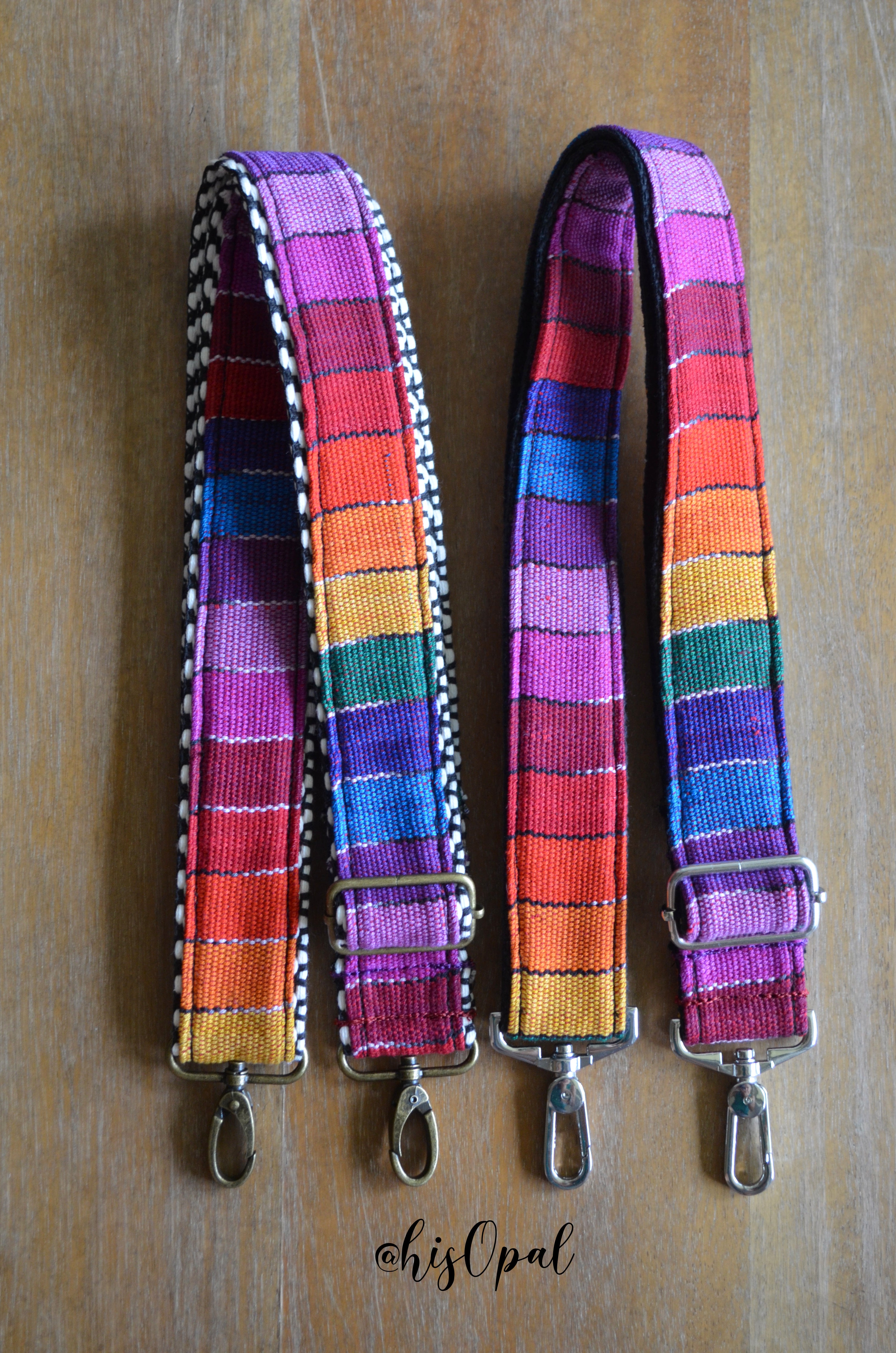This is a digital photograph of an eye-catching pair of colorful suspenders laid out on a wooden surface, with the text "his opal" written at the bottom in black. The suspenders feature a vibrant mosaic of squares in a spectrum of colors including yellow, light orange, dark orange, red, mauve, pink, purple, blue, green, and gold, making them a fun and striking accessory. Each suspender has brass clasps and pins that allow for length adjustment, and the one on the left is uniquely edged with a blue and white fringe. The suspenders likely cater to a smaller individual as they appear relatively short, but their flexibility and stretch might accommodate a variety of sizes.